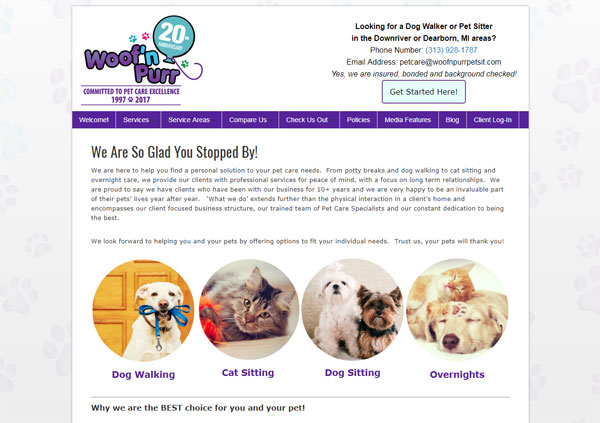Here is a more detailed and cleaned-up caption for the image:

---

The image showcases a webpage for "Wolf and Paw Pet Care," an organization renowned for its commitment to pet care excellence from 1997 to 2017. Located in the top right corner, the contact details include a phone number (313-928-1787) and an email address (petcare@wolfandpawpetsits.com), specifically for those seeking dog walking or pet sitting services in the Down River or Dearborn, MI areas. The company is highlighted as being insured, bonded, and thoroughly background-checked, offering potential clients security and peace of mind.

There is a prompt to "Get started here," guiding visitors to various links such as Welcome, Services, Service Areas, Compare Us, Check Us Out, Policies, Media Features, Blog, and Client Login. A welcoming message assures visitors of the company's dedication to helping them find personalized solutions for their pet care needs, ranging from potty breaks and dog walking to cat sitting and overnight care.